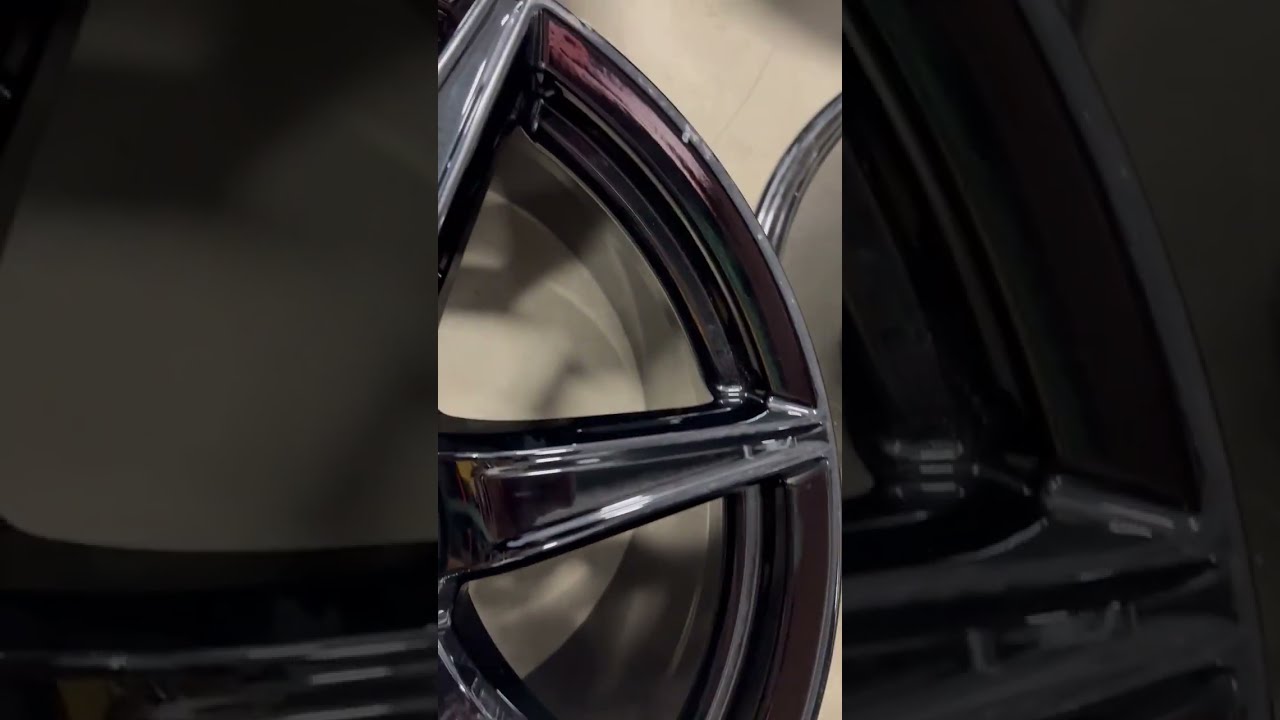The center of this horizontally aligned rectangular photo features a close-up of a chrome alloy car wheel, presented in a narrow vertical, 9 by 16 portrait orientation. This shiny silver wheel, with parts slightly reflecting a purple tint, showcases three spokes and two triangular-shaped cutouts, lending it a sophisticated metallic design reminiscent of a hubcap but with narrower and highly polished spokes. The wheel is set against a light beige or cream-colored background, which could be a tile, counter, or wall, suggesting the photo was taken indoors. The chrome wheel casts shadows on the background, enhancing its shiny appearance. The image is artistically framed by large, grayed-out, darker, and somewhat blurred sections of the wheel on both the left and right sides, creating a distinct border that draws focus to the primary subject. No people are present in the image.